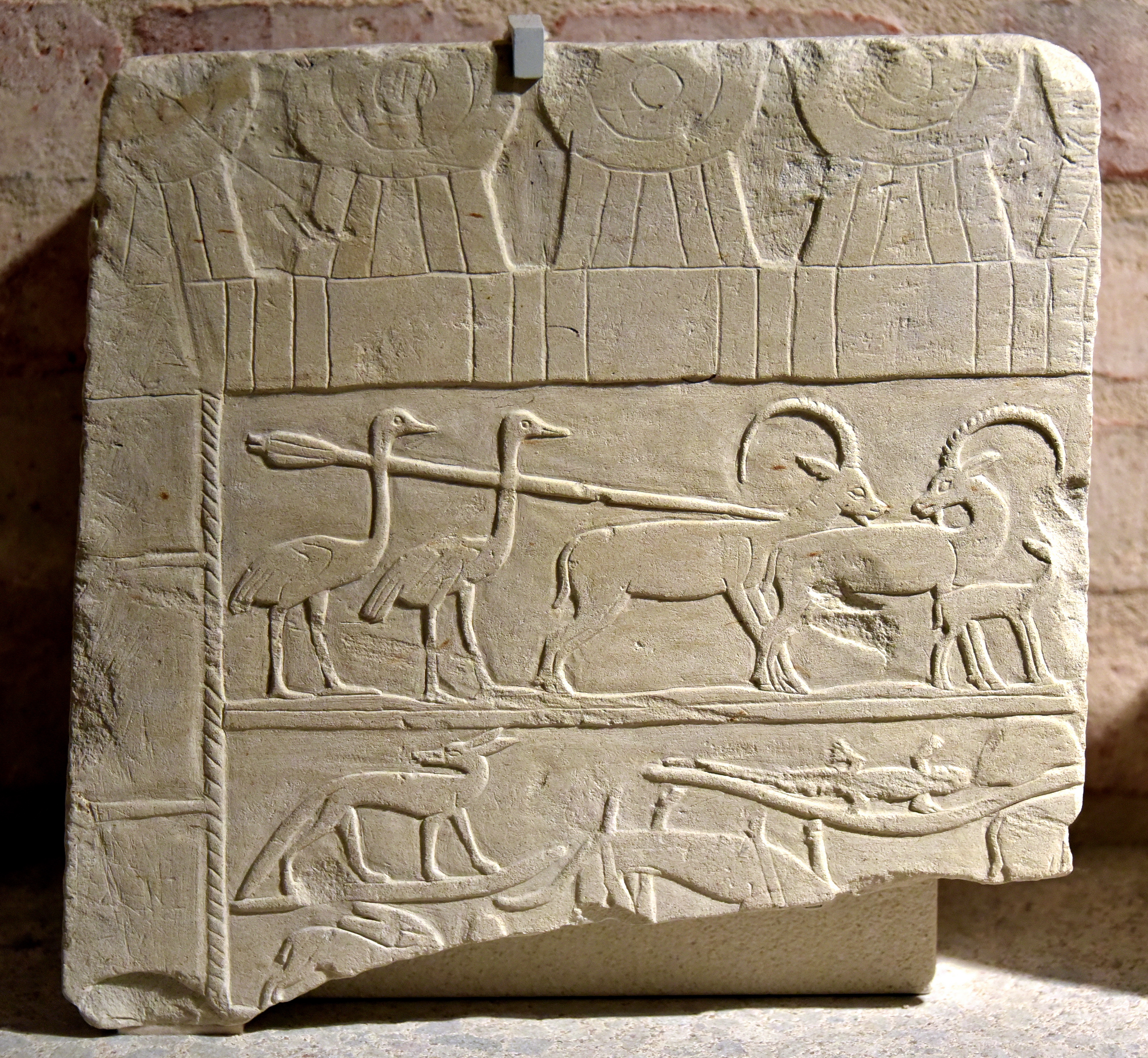In this photograph, there is an ancient, almost square-shaped stone slab of cream color, with its bottom right corner broken off on a slight diagonal from left to right. The slab features a series of intricate engravings depicting various animals. The top section of the slab shows two long-necked birds and two deer-like or goat-like animals with long, curved horns, alongside a smaller animal that could be a baby goat. A design resembling fanned shapes, similar to badminton shuttlecocks, adorns the top border. Below these figures, the middle section displays animals including a fox or wolf looking backward, a reptile, possibly a crocodile, with its head partially missing, and another reptile. The bottom section, which is broken, also features what appears to be a rabbit and possibly a lizard or another small animal. The slab is bordered by a chiselled design on the left-hand side and along the top. Behind the slab is a light peach-colored wall, and the slab itself rests on a dusty, stony floor.